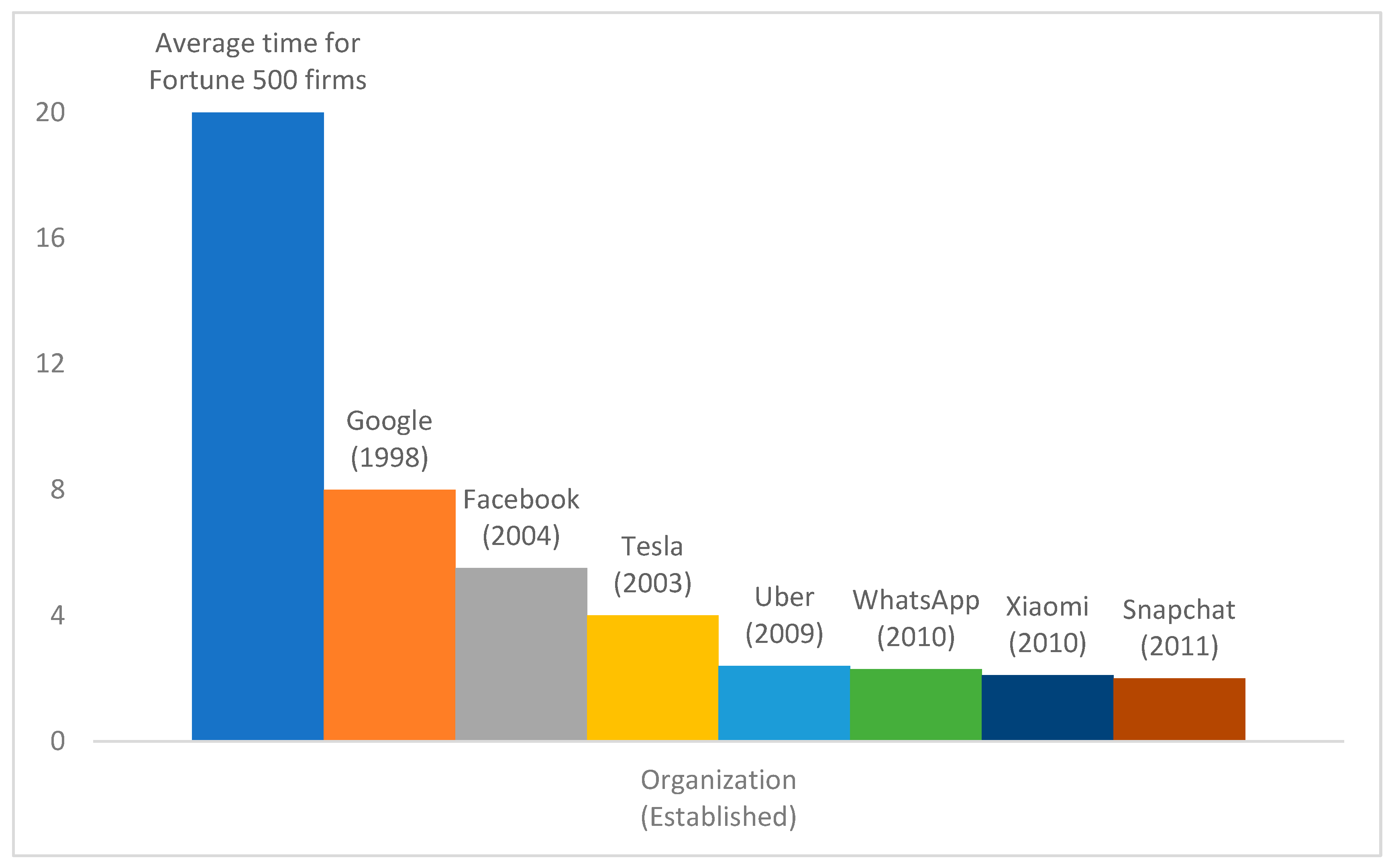This image features a detailed bar graph with a solid white background, enclosed within a black or gray square box. The vertical axis, labeled from 0 to 20 in increments of 4, represents the number of years. The horizontal axis is labeled "Organization Established" and lists various organizations by the year they were founded.

The largest bar, colored blue and nearly reaching 20, represents the "average time for Fortune 500 firms." To the right of this bar are multiple color-coded bars, each representing a different organization and its time to establishment:

1. The orange bar, marked at approximately 8, is labeled "Google, 1998."
2. The gray bar, around 6, represents "Facebook, 2004."
3. The yellow bar, near 4, indicates "Tesla, 2003."
4. A light blue bar, slightly above 3, is marked "Uber, 2009."
5. The green bar, also just above 3, is labeled "WhatsApp, 2010."
6. The dark blue bar, approximately at 3, represents "Xiaomi, 2010."
7. The brownish-orange bar, close to 3, is "Snapchat, 2011."

The bars are centrally positioned within the image, each representing the time it took for these notable organizations and others to be established, emphasizing how the average time for Fortune 500 firms compares to these more recent companies.